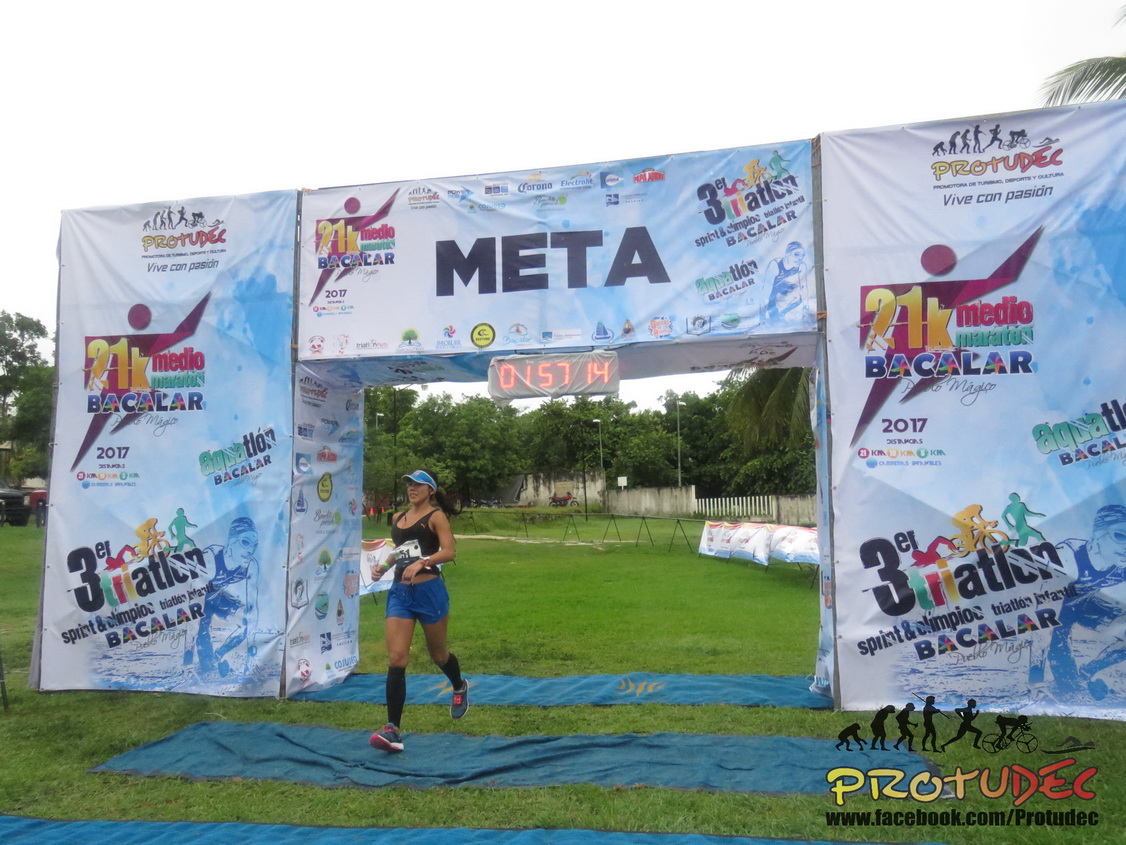In this vibrant outdoor image, a Latina woman is captured completing a half marathon under a cloudy sky. She sports blue shorts, a black crop top, and a blue visor cap, coupled with black knee-high socks and colorful blue, white, and red sneakers. She's crossing the finish line, prominently marked by a blue sign that reads "META." The backdrop features a fence, green grass, and blue tarps laid out on the ground. The finish time displayed is 1 hour, 57 minutes, and 14 seconds. The scene is peppered with various advertisements including "Pro2Dec," "21K Medio Maratón Bacalar," "Bacalar Aquatlón 2017," "Triatlón Sprint y Olímpico," "Triatlón Infantil," "Corona," and "Papa John's.” The finish line area is adorned with a distinct blue and white podium, reminiscent of clouds in the sky, enhancing the celebratory atmosphere of this athletic event.